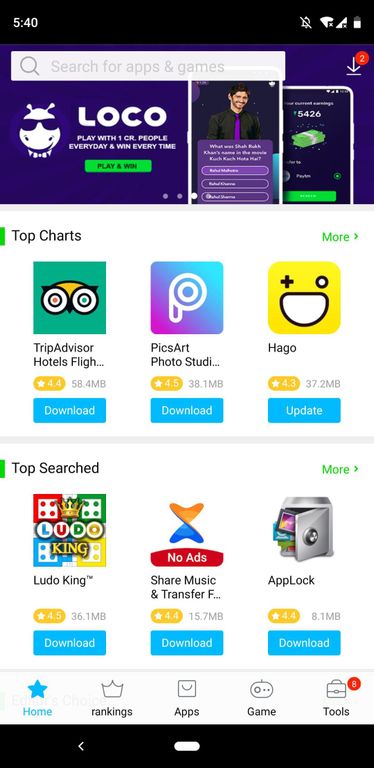**Screenshot Description:**

The screenshot features a user interface with several distinct elements and color schemes. 

- **Top Section**: A horizontal black bar runs across the top of the screen. On the left side, the current time is displayed in white. On the right side of this bar, there are icons indicating battery level, Wi-Fi signal, mobile reception, and an alarm.

- **Search Bar**: Directly below the black bar, on the left, there is a gray search bar with a magnifying glass icon on the left side. Inside the search bar, in very light print, it says, "Search for apps and games." 

- **Dropdown and Notifications**: To the right of the search bar, there is a white down arrow underlined, indicative of a dropdown menu. Above and to the right of this arrow, there is a red circle which likely denotes an alert or notification.

- **Main Content Background**: The background color changes to purple. On the left side of this purple section, there is a rectangular area featuring a company's logo. Beneath the logo, there are two lines of white text and a green button.

- **Image and Buttons**: Below the rectangle is a square image with an associated purple box at the bottom containing small white text. To the right of this, there is another square with a black background featuring a pile of green money in the center with some accompanying text.

- **Secondary Background**: Below this section, the background turns white. On the left side, there's a thin green rectangle. To the right of this rectangle, in black text, it says "Top charts." Over to the far right, "More" is written in green, accompanied by a green arrow pointing to the right, which resembles a sideways 'V'.

- **App Listing**: Below these headings, there are three horizontally-aligned rectangles, each detailing a different app:
  1. **TripAdvisor Hotels** - The app title is partially cut off (showing "F-L-I-G" after "Hotels"), with the TripAdvisor owl logo at the top and a blue download button at the bottom.
  2. **PixArt Photo Studio** - The title is partially cut off; only partially showing the "O" letter, featuring their logo at the top and a blue download button at the bottom.
  3. **HeyGo** - This app features its logo at the top and a blue "Update" button at the bottom.

- **Top Search Section**: Below this, separated by a light gray line, is the "Top search" section:
  - The layout is similar to the "Top charts" section, with the difference being that all the buttons here are labeled "Download."
  - The featured apps include LudoKing, ShareMusic and TransferF, and AppLock.